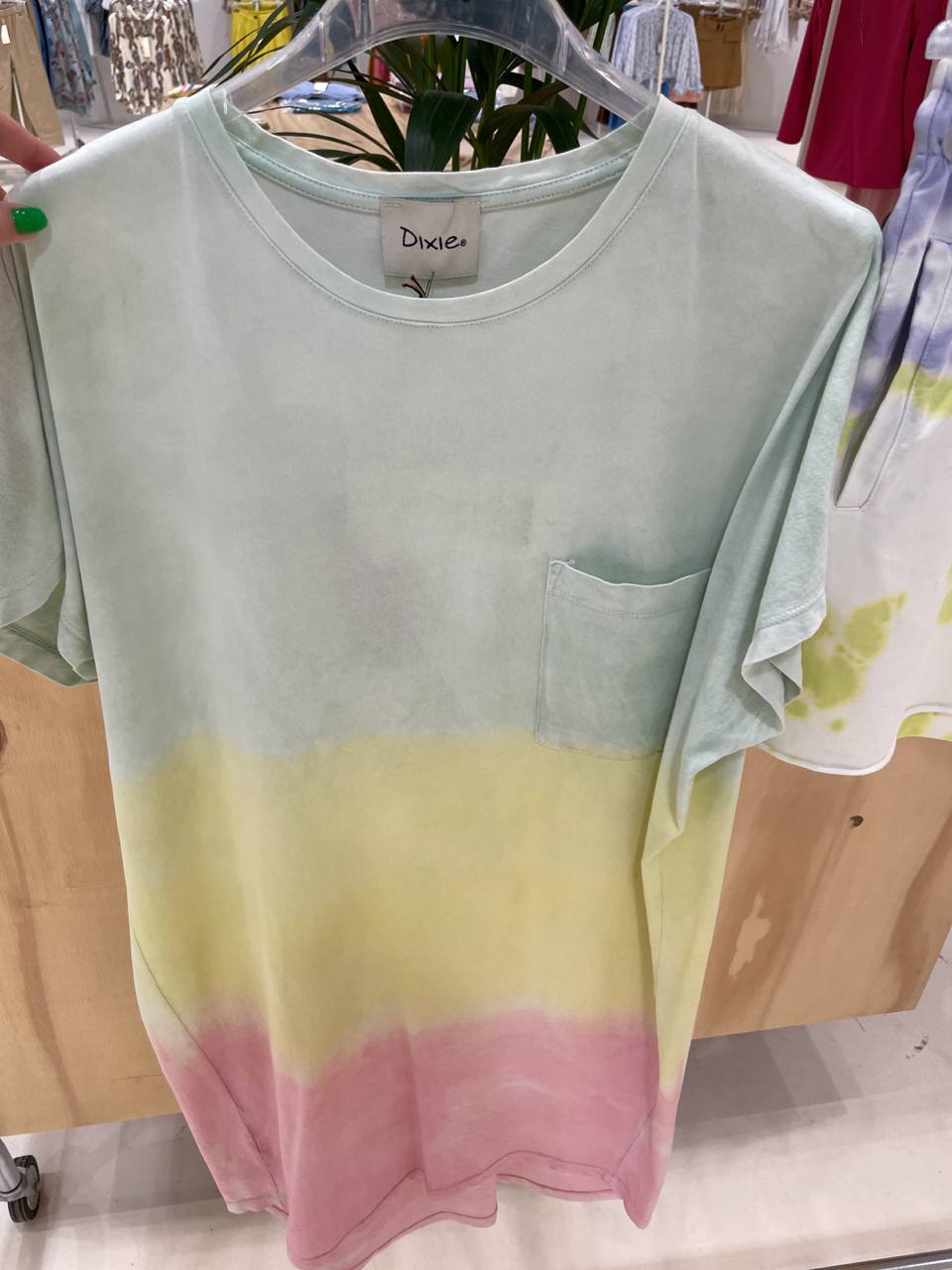This detailed photograph captures a tie-dye shirt prominently displayed in what appears to be a clothing store. The shirt, hung on a transparent plastic hanger, features a light dusty green color at the top, followed by yellow in the middle, and pink at the bottom. A small pocket adorns the chest, and a black-font label inside reads "Dixie". The shirt, slightly folded at the sleeves and bottom, hangs above a white wooden rolling bench, with shadow details and a visible wheel in the bottom left corner. To the right of the shirt, another tie-dye item, likely a pair of shorts, displays purple and green hues with a stretchy waist. On the left, a woman's hand with light skin and green-painted nails holds the shirt by the shoulder. The background showcases other indistinct clothing items and part of a green leafy plant peeking between the hanger and collar.